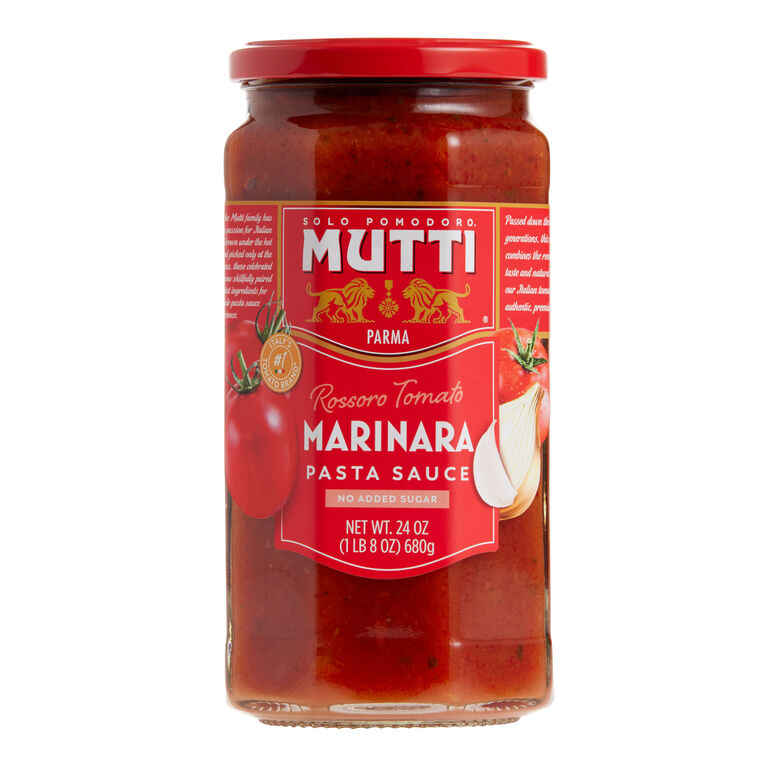This is a detailed photo of a jar of Mutti marinara pasta sauce. It features a clear glass jar, allowing a view of the vibrant red tomato sauce inside, with both lighter and darker flecks of seasoning visible. The jar has a red lid and a red label, prominently displaying a large tomato with the stem, and several cloves of garlic. The label reads "Solo Pomodoro Mutti" in white script, which translates to "Only Tomatoes Mutti," followed by "Rossoro Tomato, marinara pasta sauce." Additional text notes that there is no added sugar. Positioned between two gold lions facing each other, there is a medallion above the word "Parma." To the left of the text, there is a sticker that declares it "Italy's Number One Tomato Brand." The net weight of the jar is clearly stated as 24 ounces, or 1 pound 8 ounces, equating to 680 grams. The overall presentation emphasizes its Italian heritage and quality, with additional text possibly in both Italian and English that is partially obscured around the sides of the label.